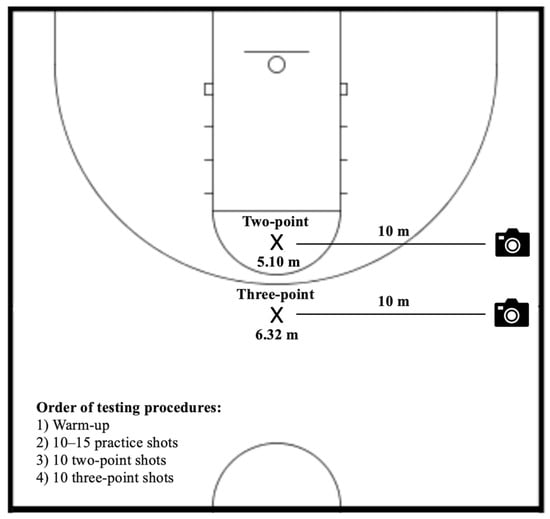The image is a square, black-and-white computer rendering of a half basketball court, viewed from an overhead perspective. The court is depicted with detailed line drawings showing the goal, backboard, lane markings, free-throw line, and the three-point arc. All dimensions are labeled in meters, such as the distance of 5.10 meters for two-point shots and 6.32 meters for three-point shots. The image features specific locations marked with Xs indicating where participants should take their shots, with additional annotations for photo spots marked by camera icons, positioned 10 meters from these points. In the bottom right corner, there is a detailed list titled "Order of Testing Procedures," outlining the steps for a workout routine or tryout: 1) Warm-up, 2) 10 to 15 practice shots, 3) 10 two-point shots, and 4) 10 three-point shots. This layout serves as a comprehensive guide for conducting and documenting the basketball shooting practice.